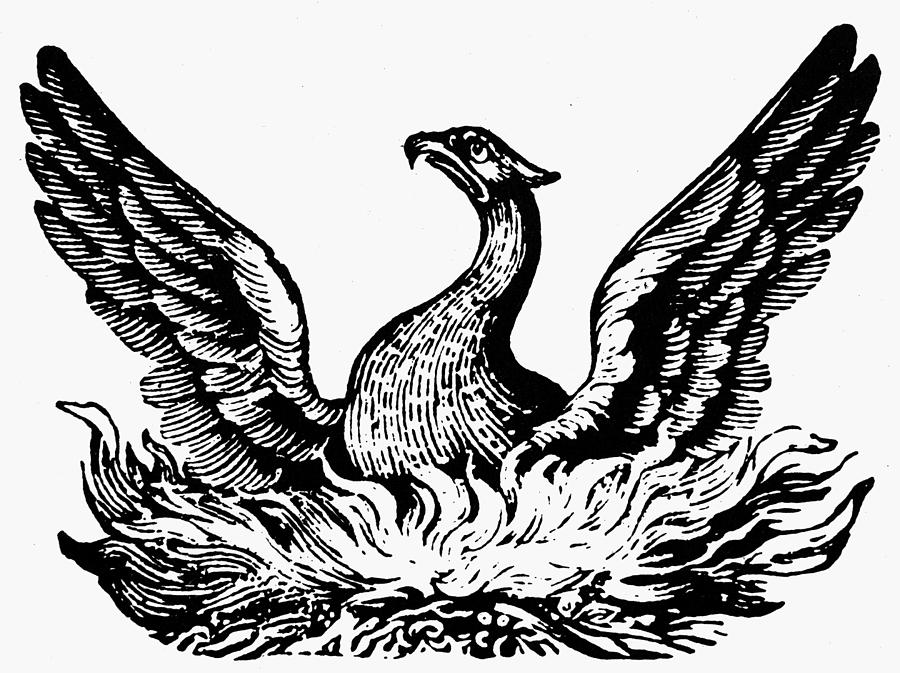The image features a detailed black and white digital drawing of a large bird, centrally positioned against a white background. The bird, which seems to be experiencing distress, is perched in a nest that some might interpret as being engulfed in flames. The bird's body is facing forward, but its head, with a notably curved neck, is turned upwards and to the left. This positioning, combined with the bird's expressive eyes, lends an air of melancholy or sadness to the scene. The wings are dramatically outstretched, reaching even higher than the bird's head, showcasing an impressive wingspan. The nest, situated at the bottom, appears to be made of grass, although the abstract, fiery lines could indicate otherwise. This artistic rendering, devoid of any text, emphasizes the bird's emotional state and the striking contrast of black lines against the stark white background.